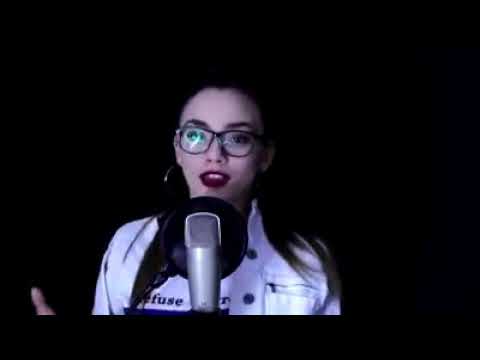The image is of a young Caucasian woman with pale skin, standing in front of a microphone against a pure black background, which is so dark that it obscures part of her hair, making it blend into the surroundings. From the chest up, she is positioned in front of a large circular microphone. The black disc of the microphone is just underneath her chin, and the rest of it is a metal gray color. The woman has straight, dark brown hair, which is pulled back into a ponytail, making her hair appear less prominent. She has finely arched dark brown eyebrows and wears dark, large-rimmed glasses. Her eye makeup is noticeable, possibly including false eyelashes. She has prominent red lipstick that is almost the darkest shade of red. She's dressed in a white denim jacket over a white t-shirt that has some black text on it, partly visible as the letters F-U-S-E. One of her hands is slightly raised, indicating that she is in the middle of speaking when the photo was taken. The entire image is framed by black bars on the top and bottom, with the bottom bar notably cutting off part of her body.